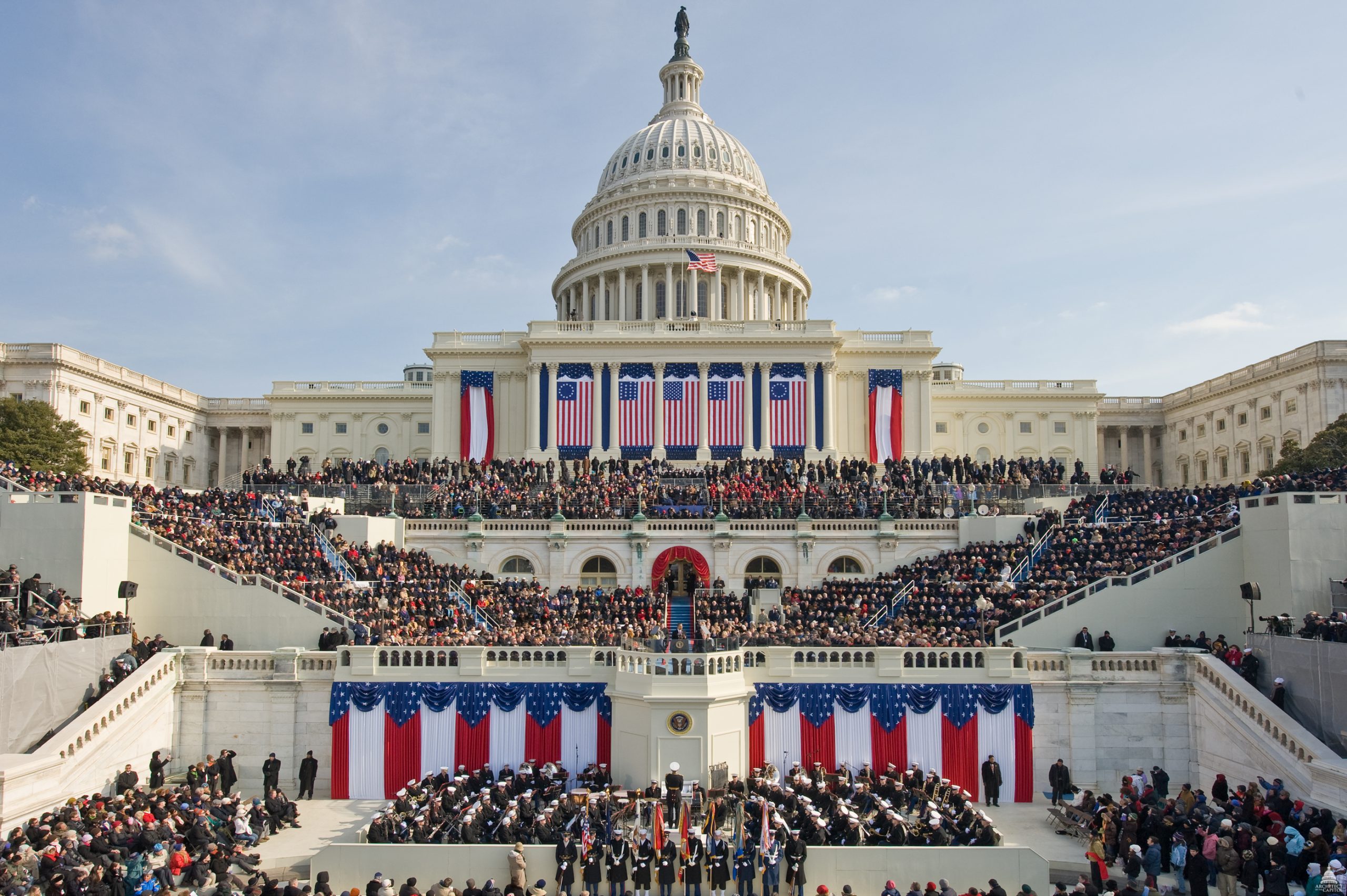This detailed photograph captures the United States Capitol building against a backdrop of a blue sky with light cloud cover, indicating the event is taking place outdoors. The iconic structure is adorned with numerous American flags and extensive red, white, and blue decorations, suggesting a patriotic celebration, possibly an inauguration. The scene is densely packed with people filling every available space, from the grand staircases to the various balconies. At the forefront, a military band accompanied by a color guard stands ceremoniously before a sea of attendees. Central to the image is a podium, presumably where the President or another high-profile politician is delivering a speech. The entire atmosphere exudes a sense of national pride and monumental significance.